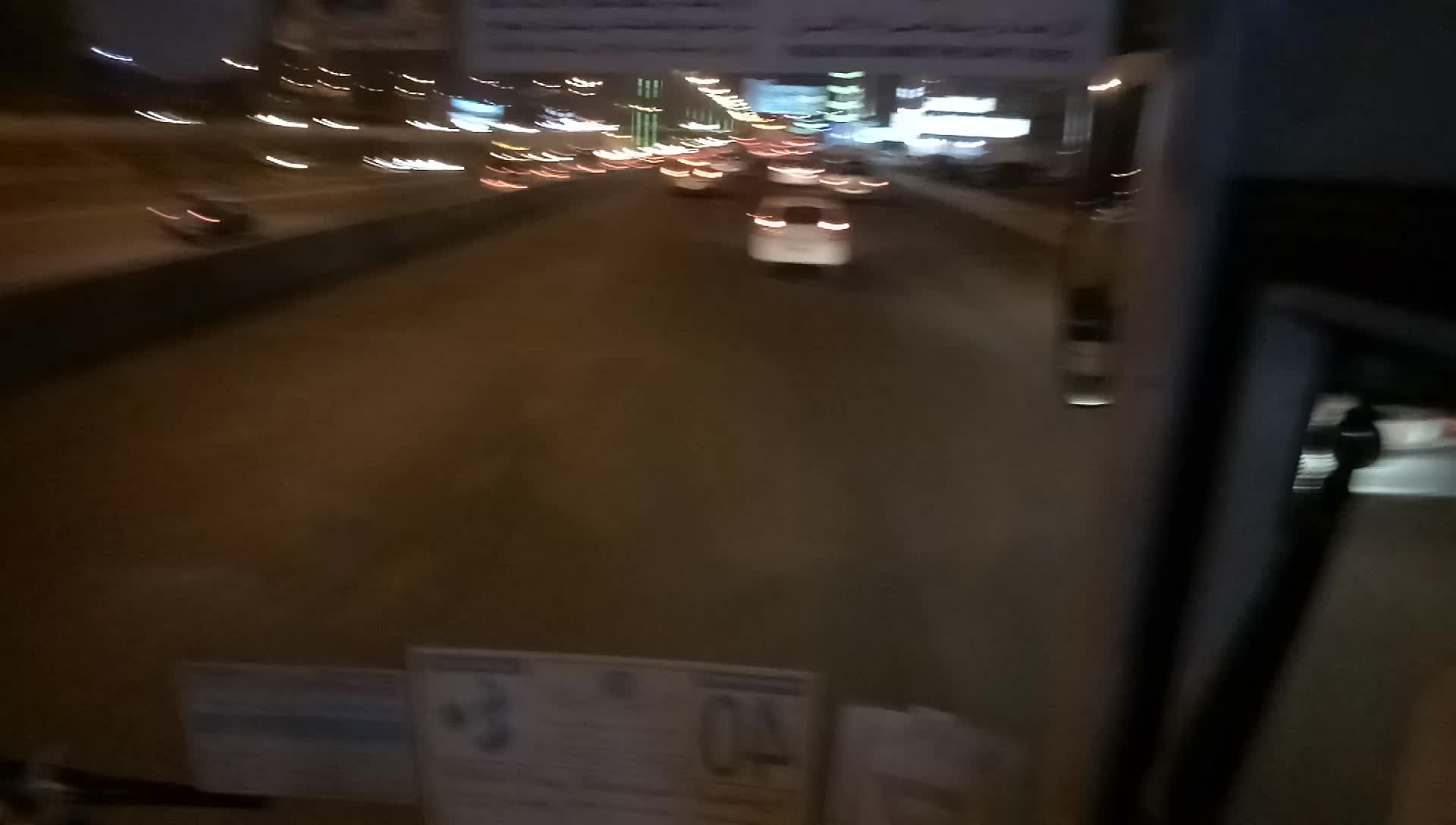In this very blurry nighttime image taken through the large front windshield of a bus, we're given a view of a busy interstate with three lanes. The photograph, marked by reflections of leaflets or papers at the bottom, illustrates a scene slightly obscured by window stickers in the bottom right corner, notably one depicting the number 40. Hanging signs are visible above the windshield, along with a doorway to the right, highlighting the bus's sizable interior. A white car with somewhat pale brake lights is immediately in front of the bus, trailed by dimly lit taillights of other vehicles on the same road. To the left, separated by a concrete barrier, another three lanes of traffic head in the opposite direction, illuminated by the headlights of oncoming cars. Additional details include a large, dark grey object with discernible poles and sections, street lights, and distant building lights contributing to the nighttime ambiance. There is also a bright white rectangular sign in the upper right portion of the photo and an Interstate sign visible farther ahead, subtly hinting at the urban backdrop.